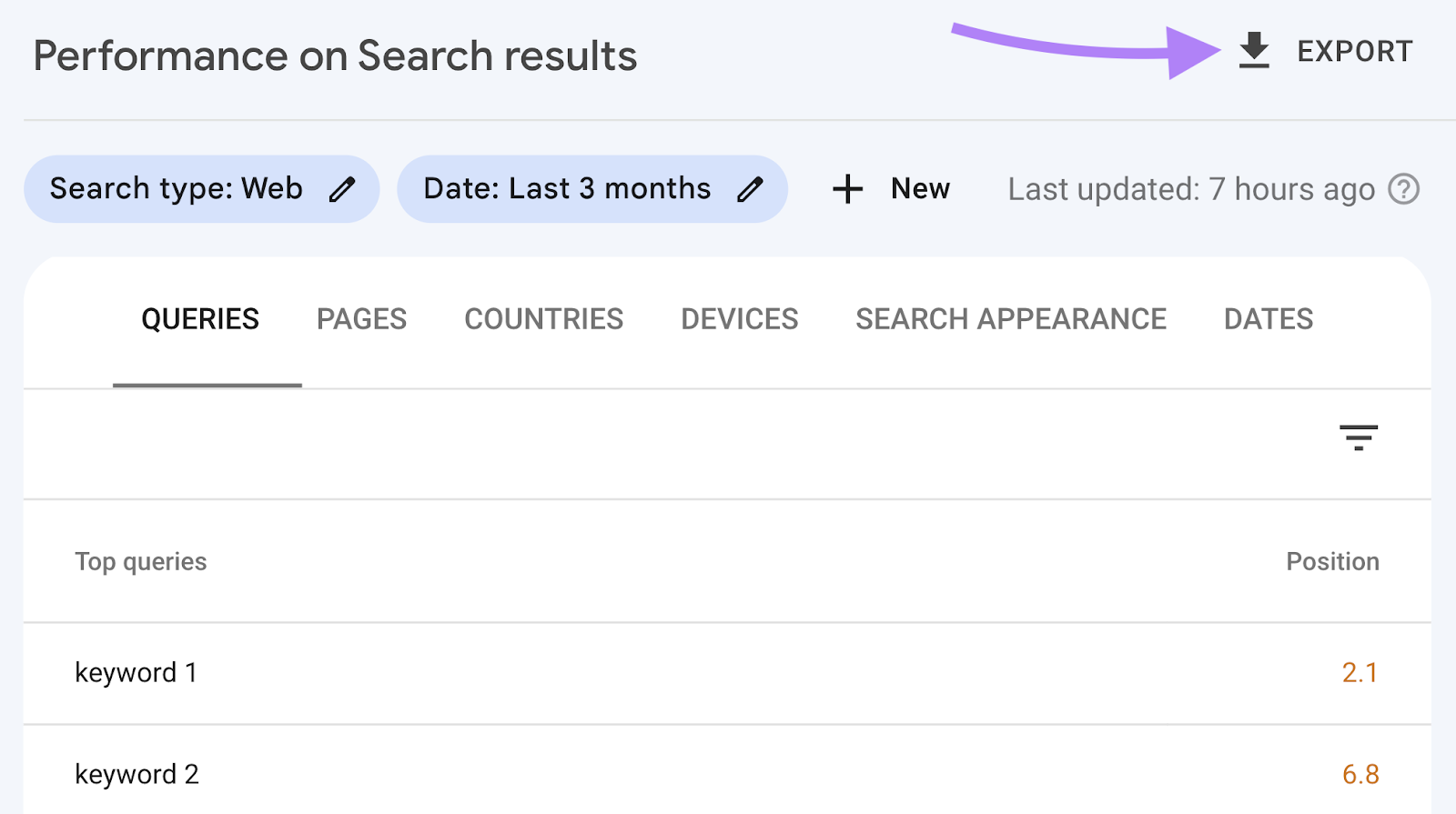The image depicts a rectangular interface, wider than it is tall, which appears to be a screenshot from a web analytics tool focused on performance metrics for search results. 

In the upper left corner, the text "Performance on search results" is prominently displayed in black. On the upper right side, there is an icon indicating a download option with a downward arrow next to the word "Export." A purple arrow, likely added by a photo editor for emphasis, points directly at the export option, suggesting its importance, possibly for educational purposes.

A gray line separates the top section from the main content area. Below this line, there is a button labeled "Search type: Web" with an editable pencil icon next to it. Another editable pencil icon, colored blue, appears next to the date range "Last 3 months." Following this are indicators for adding new filters or settings, such as a plus sign and the text "New," accompanied by the statement "Last updated 7 hours ago." A question mark inside a circle is also visible, typically signaling the presence of help or more information.

Further down, a navigation bar with tabs for different metrics categorizes the data: "Queries," "Pages," "Countries," "Devices," "Search Appearance," and "Dates." The "Queries" tab is selected and highlighted in black with a black underline, whereas the other tabs are in gray.

Under this navigation bar, another line appears. To the right of this line is a triangle icon made of three horizontal black lines pointing downward. The next line denotes "Top Queries," with "Position" aligned to the right.

Below this header, a list of search queries and their respective positions is displayed. The first entry, "Keyword 1," has a position of "2.1" highlighted in red on the right. The second entry, "Keyword 2," shows a position of "6.8," also in red.

This meticulous breakdown offers a clear understanding of a tool designed to measure the performance of specific search queries over a designated timeframe.